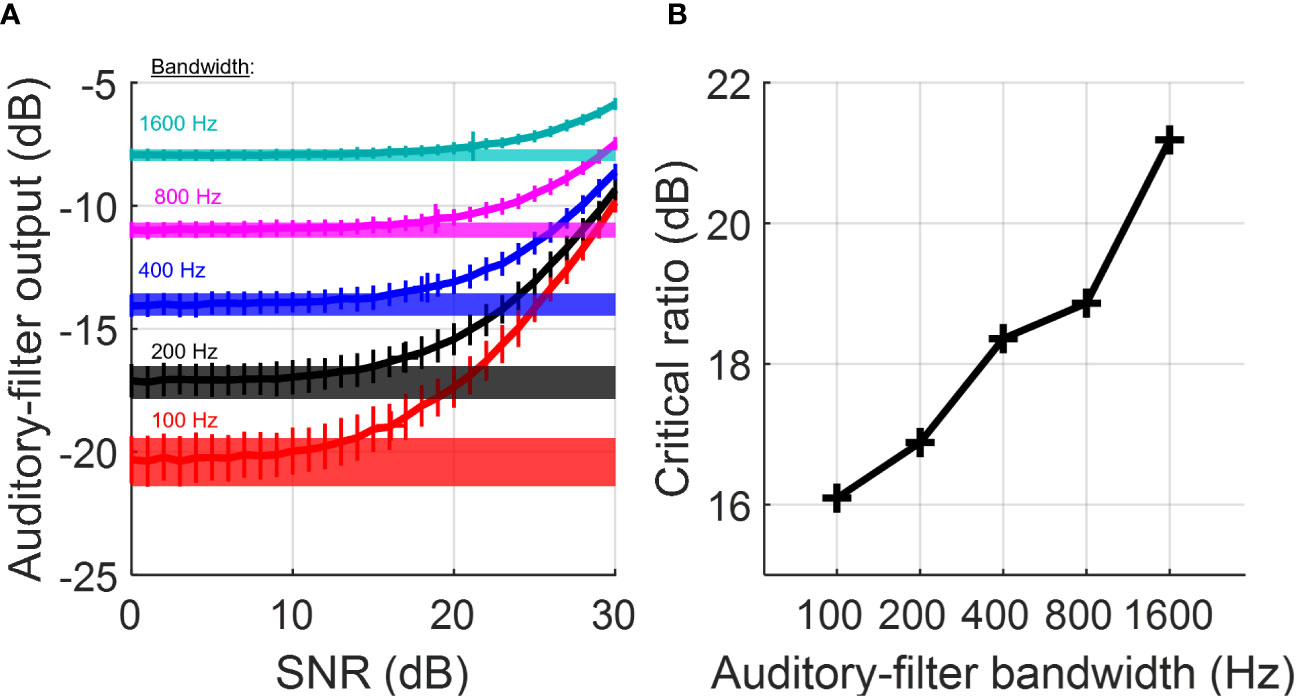This color photograph features two side-by-side graphs that illustrate auditory filter analyses. 

On the left, Graph A is a line graph titled "Auditory Filter Output (dB)." The vertical axis measures decibels (from -25 to -5), and the horizontal axis measures Signal-to-Noise Ratio (SNR) in decibels (from 0 to 30). It has five distinct horizontal lines, each representing different frequencies: solid red at -20 dB for 100 Hz, solid black at -17.5 dB for 200 Hz, solid blue at -15 dB for 400 Hz, solid purple at -10 dB for 800 Hz, and teal at -7.5 dB for 1600 Hz. These lines arc upward and to the right, resembling railroad tracks. 

On the right, Graph B is a bar graph depicting the "Critical Ratio (dB)" against "Auditory Filter Bandwidth (Hz)." The vertical axis shows decibels (from 16 to 22), while the horizontal axis presents bandwidths (100, 200, 400, 800, and 1600 Hz). The graph has six upward plots connected by a solid black line, starting from 100 Hz at 16 dB and rising to 1600 Hz at just above 21 dB.

Both graphs are detailed with different colors—red, black, blue, purple, and green—highlighting the various Hertz measurements and their corresponding decibel levels. Together, these graphs visually represent how auditory filter output and critical ratios vary with changes in frequency and bandwidth.